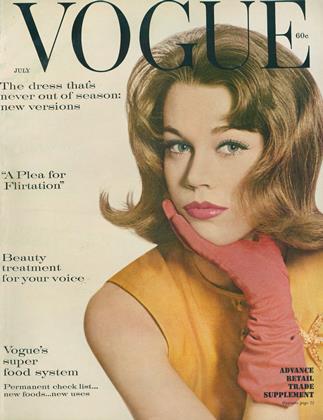The image is the cover of the July 1st, 1959 issue of Vogue magazine, priced at $0.60. The cover features a high-fashion photograph of Jane Fonda, who poses elegantly with her hand resting on her chin, wearing an orange sleeveless top and pink gloves. Jane, a white woman with auburn, almost light brown hair, and green eyes, is adorned with red makeup and lipstick. The background of the cover is tan, and the text is black. Prominently featured articles on the cover include "The Dress That's Never Out of Season," "New Versions," "A Plea for Flirtation," "Beauty Treatment for Your Voice," "Vogue's Superfood System," "Permanent Checklist," "New Foods," "New Issue," and "Advanced Retail Trade Supplement."